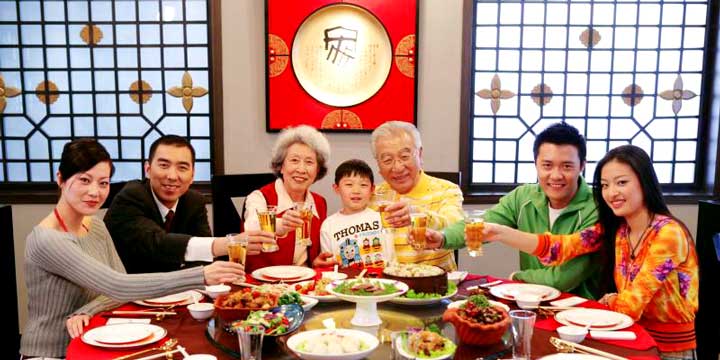This full-color photograph captures a joyful family meal in an Asian restaurant, rendered in a horizontally rectangular frame without a distinct border or background. Centrally placed around a red table laden with food, a large family of Asian descent smiles and toasts with glasses of a yellowish-amber liquid, possibly beer. Everyone is facing the camera, sharing a festive moment together. 

In the center of the image stands a young boy wearing a white t-shirt featuring "Thomas the Tank Engine," with the character's blue train image and gray face prominently displayed. Flanking the boy are an elderly woman in a white collared shirt and red vest on the left, and an elderly man in a yellow and white shirt on the right. To their sides, on the far left, a man in a black suit and tie and a woman in a gray long-sleeved shirt appear to be in their 30s or 40s. On the far right, a younger man in a green collared shirt and a younger woman in an orange shirt are possibly in their 20s or 30s.

The background features two large, opaque windows with grid designs and decorative plus signs and circles in the upper left and right corners. In the top center, a red square with a white circle and Asian writing adds a cultural touch to the setting, indicating the festive atmosphere within the restaurant. The photograph perfectly encapsulates a candid and warm family gathering.